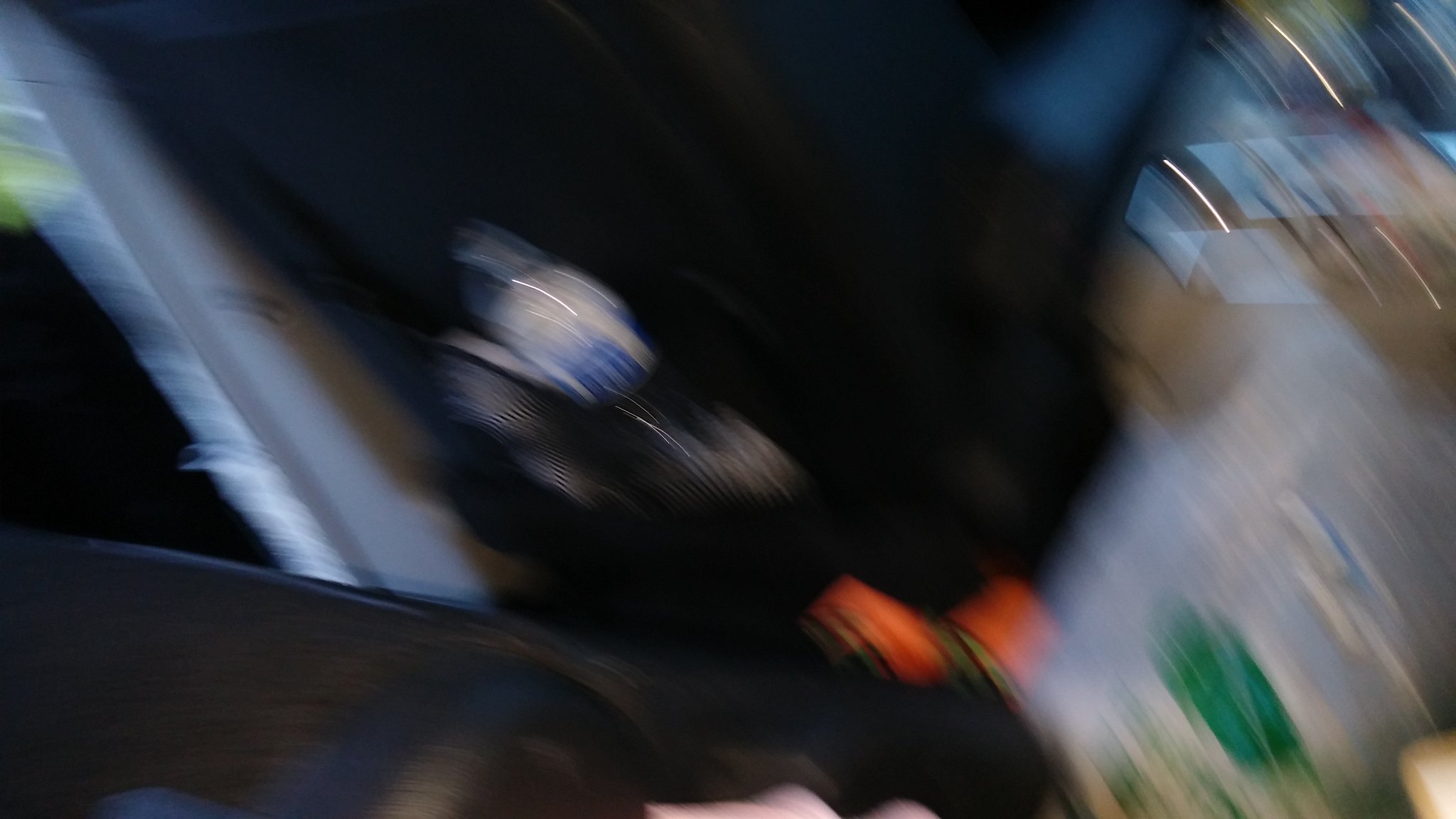This image is an extremely blurry and heavily distorted color photograph that seems to capture an indiscernible scene. Blurs and ghosted shapes dominate the frame, suggesting multiple items overlaid on each other. The overall dark ambiance implies it may have been taken at night or underexposed, perhaps even accidentally with a smartphone. On the left, a solid object resembling the bottom of a boat or yacht stands out, while towards the right, there might be a disposable carrier bag with some green logos. The center appears to have a vague shape of a water bottle within a black object, among what might be leather or fabric elements, potentially indicating the inside of a car with a center console visible. Scattered across the scene, there are indistinct boxes, possibly brown with white labels and some gold accents, and vague orange items on the ground. Reflective lines add to the confusion, making it almost impossible to discern the exact content or context of the photograph.